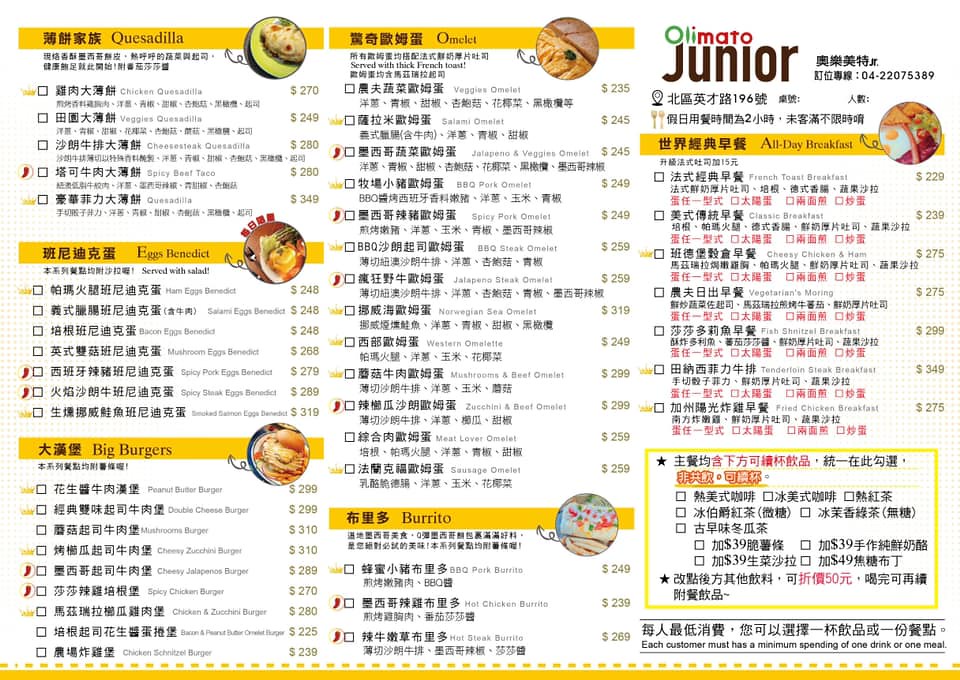This image depicts a Chinese menu filled with numerous items listed in both Chinese and English. The menu is organized into three columns, each topped with a yellow horizontal line that categorizes different sections. The sections are annotated with Chinese characters followed by their English translations. Among these sections, notable headers include "Quesadilla," "Omelet," "Eggs Benedict," "Big Burgers," "Burrito," and "All Day Breakfast."

In the top rightmost column, the word "Olimato" is conspicuously displayed, spelled out in striking green and red letters, while the word "Junior" is directly underneath in brown letters. 

Each yellow header line also incorporates a small, colorful image of a food item, providing a visual cue for the respective section. The menu items are accompanied by prices, each preceded by a dollar sign. Notably, there are no decimals in these prices, which are all three digits; for example, the "Meat Lover Omelet" is marked at $259, presumably $2.59.